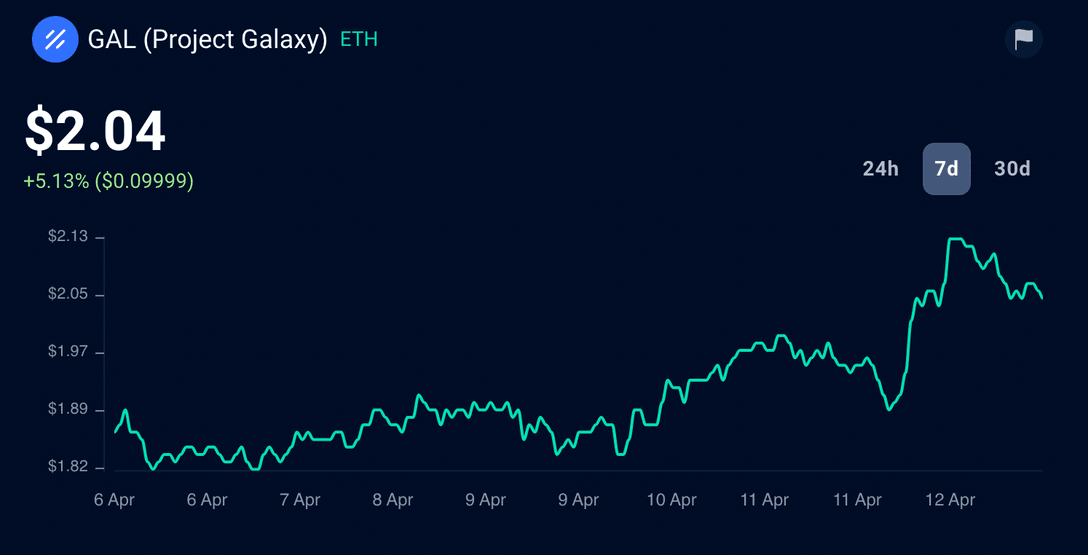The screenshot depicts a horizontal chart from a mobile device featuring a jet-black background. The chart is titled "GAL (Project Galaxy) - ETH," suggesting it represents the cryptocurrency Project Galaxy in relation to Ethereum. To the left of the title, there is a logo consisting of a blue circle with three diagonal white lines.

The current price of GAL is prominently displayed in bold white font at $2.04. Below the price, it indicates a positive change with a value of +5.13% (0.09999). The vertical axis on the left side of the chart is labeled with the following price markers from top to bottom: $2.13, $2.05, $1.97, $1.89, and $1.82. The horizontal axis at the bottom shows date markings: two instances of April 6, and one instance each for April 7, April 8, April 9, April 10, April 11, and April 12.

In the upper right-hand corner of the screenshot, there is a flag icon. The chart represents a 7-day period and is characterized by a thin green line that indicates a noticeable rise in the value of the cryptocurrency GAL over the specified timespan.